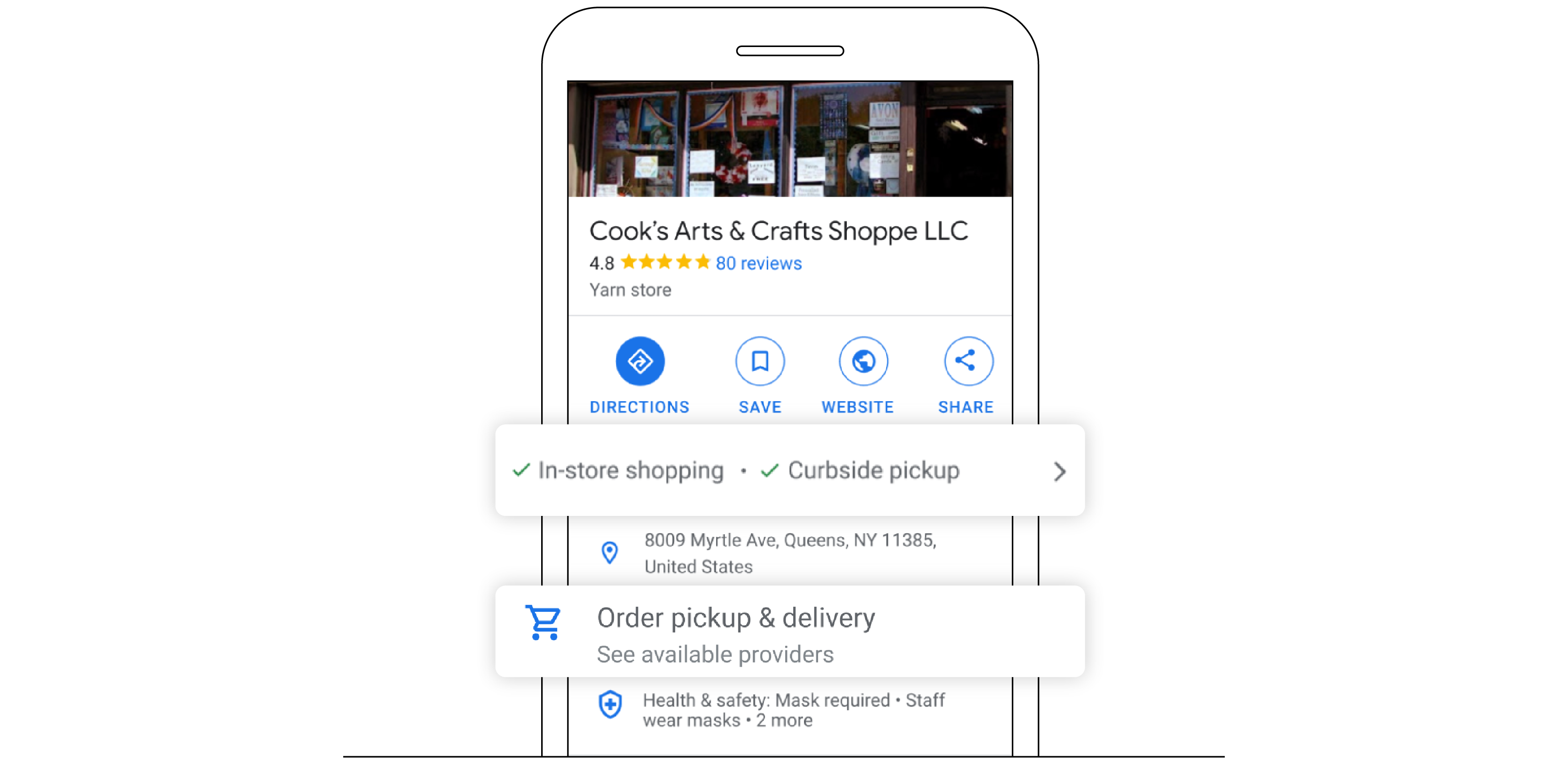A stylized digital representation of a mobile phone screen displays a Google search snippet for "Cook's Arts and Crafts Shop, LLC." The diagram features the upper half of a phone, with the search results superimposed onto the screen, giving the illusion that this information is being viewed on a phone. The business highlighted is "Cook's Arts and Crafts Shop," located at 8009 Myrtle Avenue, Queens, New York. The shop boasts a Google rating with 80 reviews. The image also includes icons for navigating to the business, visiting its website, sharing its details, and saving the information for later.

An inset photo, presumably showing the exterior of the shop, is too small to discern specific details but adds a visual touch to the listing. Health and safety information indicates that both customers and staff are required to wear masks. Furthermore, the business offers several convenient options such as store pickup, delivery, in-store shopping, and curbside pickup, all clickable for additional details. The minimalist white background of the diagram ensures that all textual and visual elements stand out clearly.